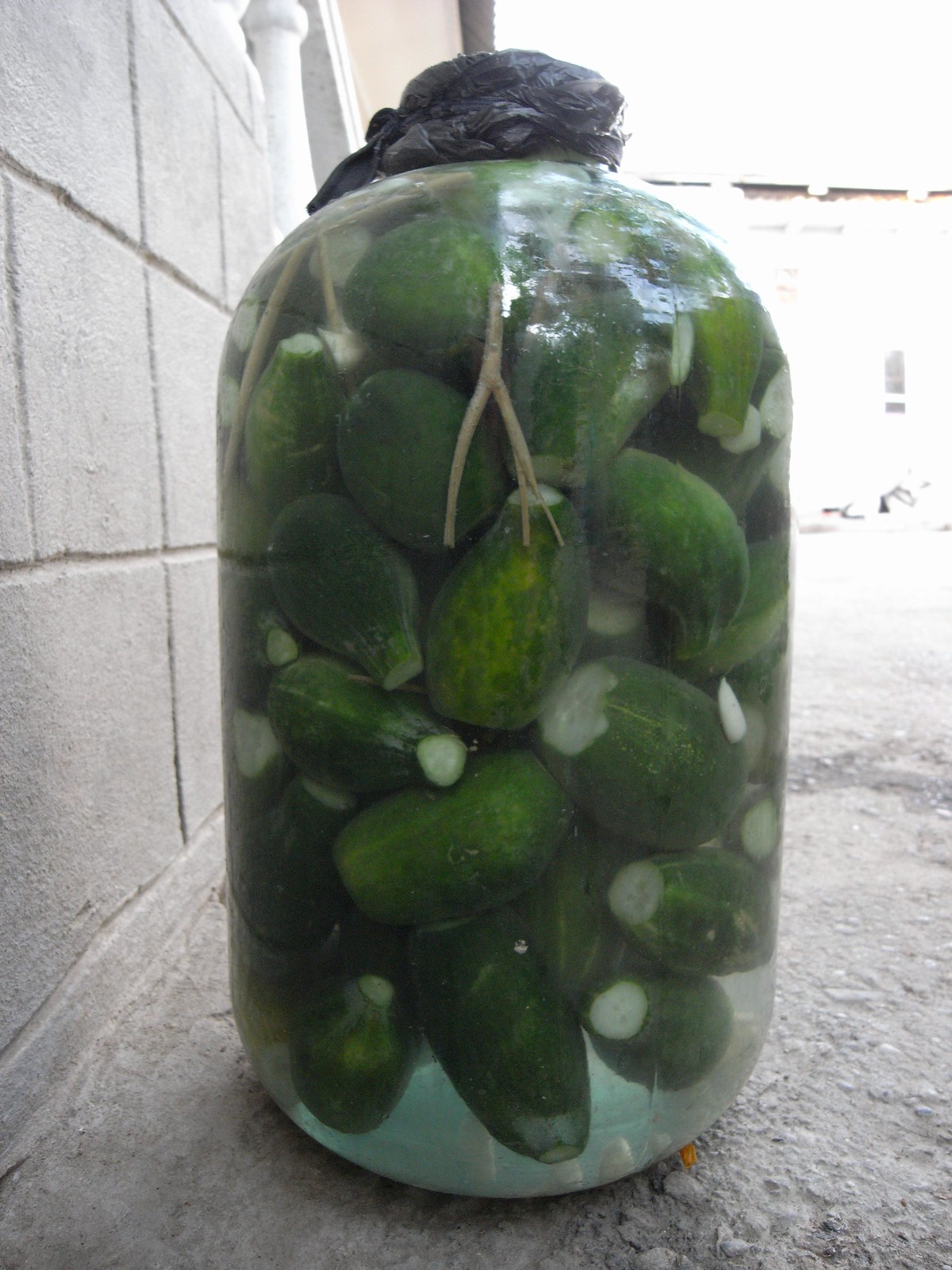In this image, a close-up view of a large glass jar is shown resting on the ground outside against a concrete wall. The jar contains green, avocado-sized fruits that are pointed at one end and white at the tips, resembling stubby cucumbers. These fruits are submerged in a clear liquid, alongside floating garlic-like white pieces and a few slender sticks or twigs, which could be seasoning agents. The lid of the jar is covered with a black plastic bag, secured around the top. The background is extremely bright, with sunlight washing out most details, but a gravelly, rocky ground, and elements of a stone wall and white pillars can be faintly discerned.